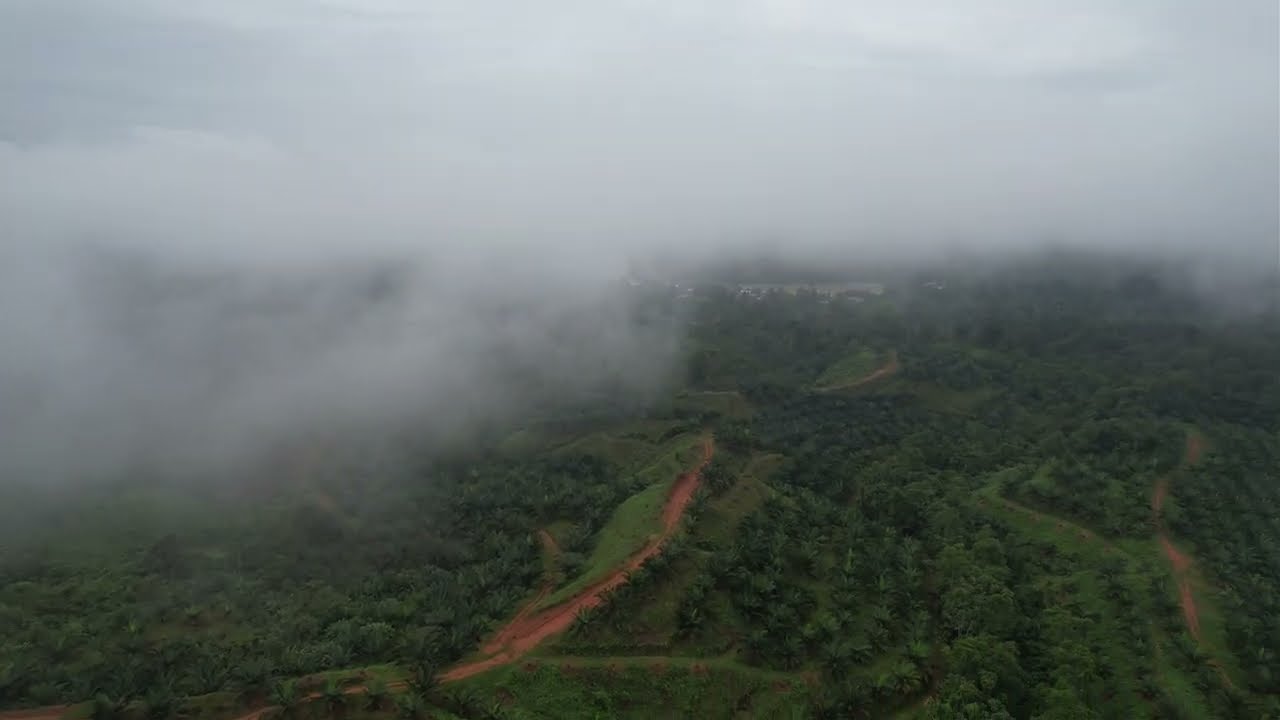This aerial photograph, likely taken from a low-flying plane or helicopter, captures an expansive and predominantly green landscape dominated by rows of lush trees and bushes. The verdant scene extends horizontally from left to right and reaches deep into the background. Two prominent dirt roads meander through this greenery; one originates from the lower left corner and curves upwards toward the center, continuing into the distant horizon, while another starts at the lower right corner, cutting through an array of trees. A low-hanging cloud occupies the center-left portion of the image, blending with the overcast white sky, making the boundary between cloud and sky almost indistinguishable. Additionally, fog blankets parts of the ground, especially the left and background sections, enhancing the cloudy and overcast ambiance of the day. Apart from the natural elements, no human structures are visible, suggesting the scene might be a vast farmland or a dense countryside.